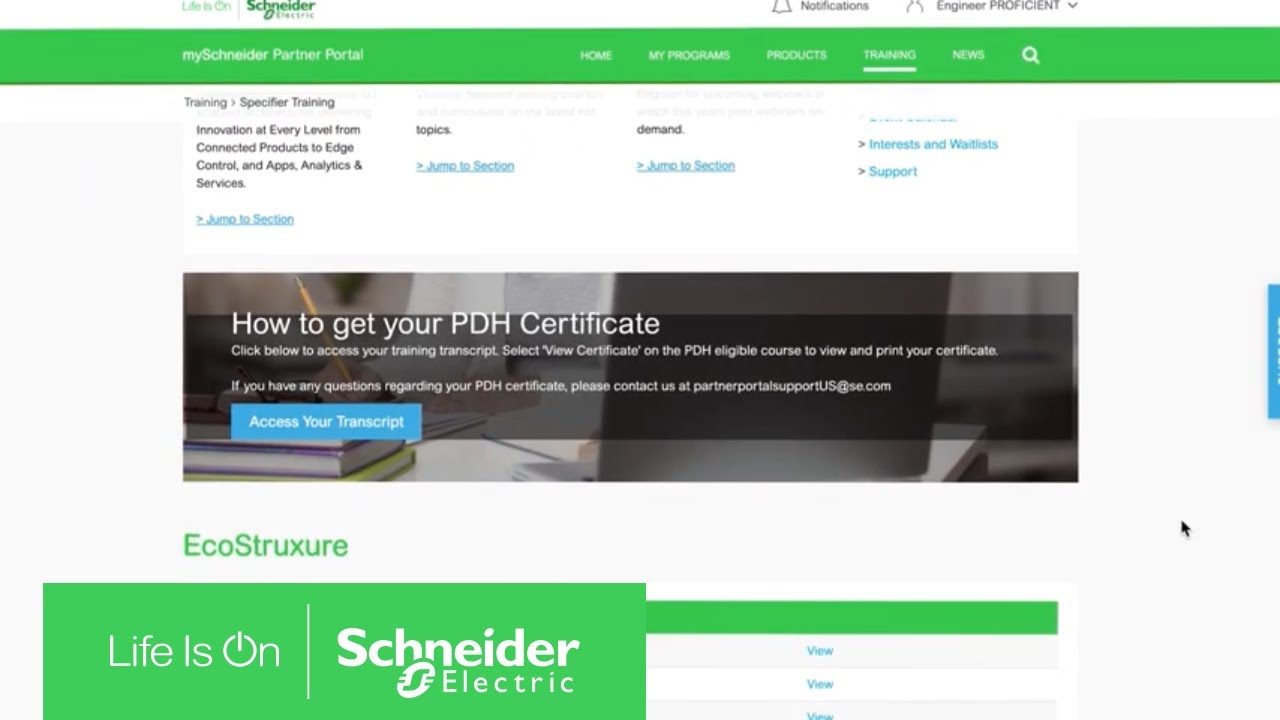**Homepage Overview of Schneider Electric's mySchneider Partner Portal**

At the top of the page, there is a green banner displaying the text "Life is On" followed by a vertical line and "Schneider Electric" in small font. Towards the right of this banner, there's an icon for notifications and a profile section labeled "Engineer Proficient" with a dropdown arrow for more options.

Below the green banner, there's a long green rectangular tab with white text that reads "mySchneider Partner Portal." Continuing across to the right, the navigation menu includes links labeled "Home," "My Programs," "Products," "Training" (highlighted with a white underline indicating it's the current section), "News," and a magnifying glass icon for search.

The main content area of the page is headed by the title "Training" followed by a descriptive arrow. The page includes several sections of small black text that are difficult to read and each section is accompanied by blue hyperlinked text, presumably for navigating to different sections.

There is a rectangular image on the page, featuring books and a person writing. Overlaying this image is the text "How to Get Your PDH Certificate," along with a couple of lines of smaller text and a blue button labeled "Access Your Transcript."

Below this image, in green text, is the word "EcoStruxure." Further down, there's another green rectangular banner with the text "Life is On" followed by a line and "Schneider Electric" in white text.